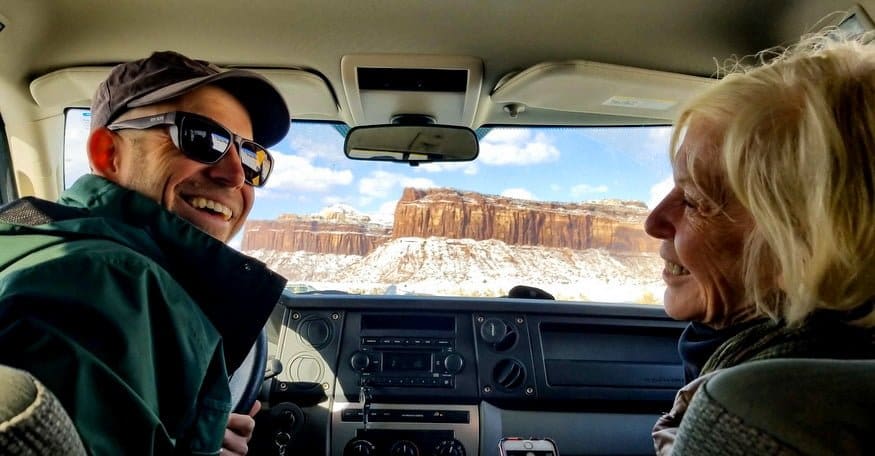The photograph, which is in landscape layout, captures a man and a woman inside a car with a light tan interior. The man, seated in the driver's seat, is turning back to smile at the camera. He is wearing a brown cap, sunglasses, and a green jacket, and appears to be Caucasian. The woman in the passenger seat, also Caucasian, has blonde hair and is smiling while wearing a green and blue sweater. The image is taken from the backseat, providing a view of the dashboard, which is black, and the tan-colored ceiling of the car. Through the front windshield, a stunning snowy landscape can be seen, featuring the Grand Canyon or a similar reddish rocky terrain with a clear blue sky and scattered white clouds above.